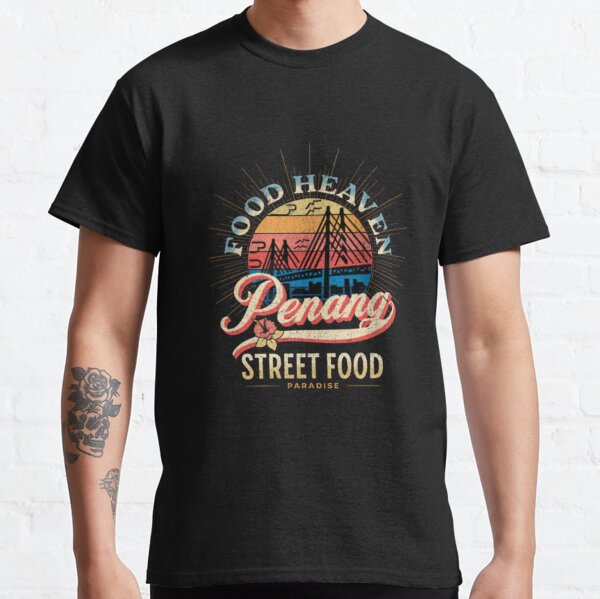The image features a male model, shown from the neck down to the top of his waist, wearing a black crewneck t-shirt. The t-shirt prominently displays a circular logo with horizontal stripes in red, yellow, gold, and pink. At the top of the circle, it reads "Food Heaven" in blue and pinkish lettering, with sun rays emanating above the text. Within the circle, there is an illustration of a large bridge, resembling the Golden Gate Bridge, against a sunset backdrop. Below the bridge, the word "Penang" is written in a cursive style with an elaborate ‘G’ that extends beneath the word. Further down, the phrase "Street Food Paradise" is inscribed, with lines separating "Street Food" and "Paradise." Additionally, the model has two visible tattoos on his right arm: one on his forearm, depicting a detailed design that could be interpreted as a skull with flowers and possibly a monkey face, and another, less discernible tattoo on his wrist. The subject of the photo appears to be either Caucasian or Hispanic.